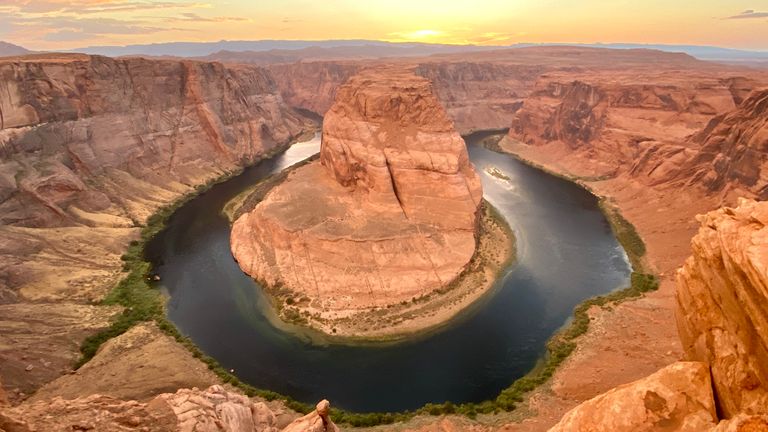This image captures the iconic Horseshoe Bend, a breathtaking natural feature located in the Arizona-Utah area, part of the Colorado River. Dominating the scene is a massive butte formation, encircled by the river that flows from the upper left, curving gracefully around the bend, and continuing to the upper right. The water is dark and murky, with green growth lining the banks where it meets the rock. The surrounding landscape features striking red rocks, exhibiting a palette of creams, tans, and browns, enhanced with natural lines and bulges that add character to the terrain. The flatness of the foreground extends to distant, slightly undulating hills. The sky is partly cloudy, with sunlight piercing through the center, adding a glowing ambiance to this beautifully elongated photograph. This iconic spot, often likened to the grandeur of the Grand Canyon, is a popular tourist destination, enticing many to capture its splendor.